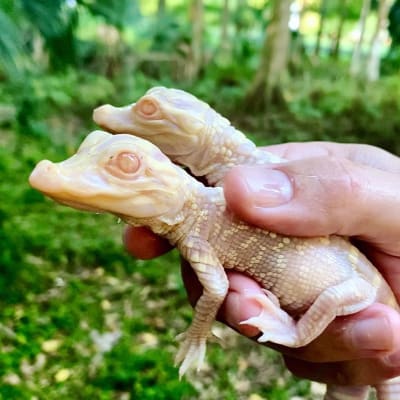In this detailed and vivid photograph, a human hand is prominently featured holding two incredibly young, almost albino alligators or possibly crocodiles, each showing very pale, translucent skin that diverges between a whitish-yellow hue and a human-like neutral tone. These tiny reptiles, likely just a day or two old, display underdeveloped eyes with barely distinguishable pupils and have little yellow specks and dots signifying the early stages of scale formation. They are also equipped with webbed feet. The image is taken outdoors, set against a lush, verdant backdrop that almost resembles a jungle or swamp, filled with vibrant green vegetation and indistinct, out-of-focus trees, possibly cypress. The natural setting enhances the delicate, new life of these barely hatched reptiles, capturing a serene, almost magical moment in nature's cycle.